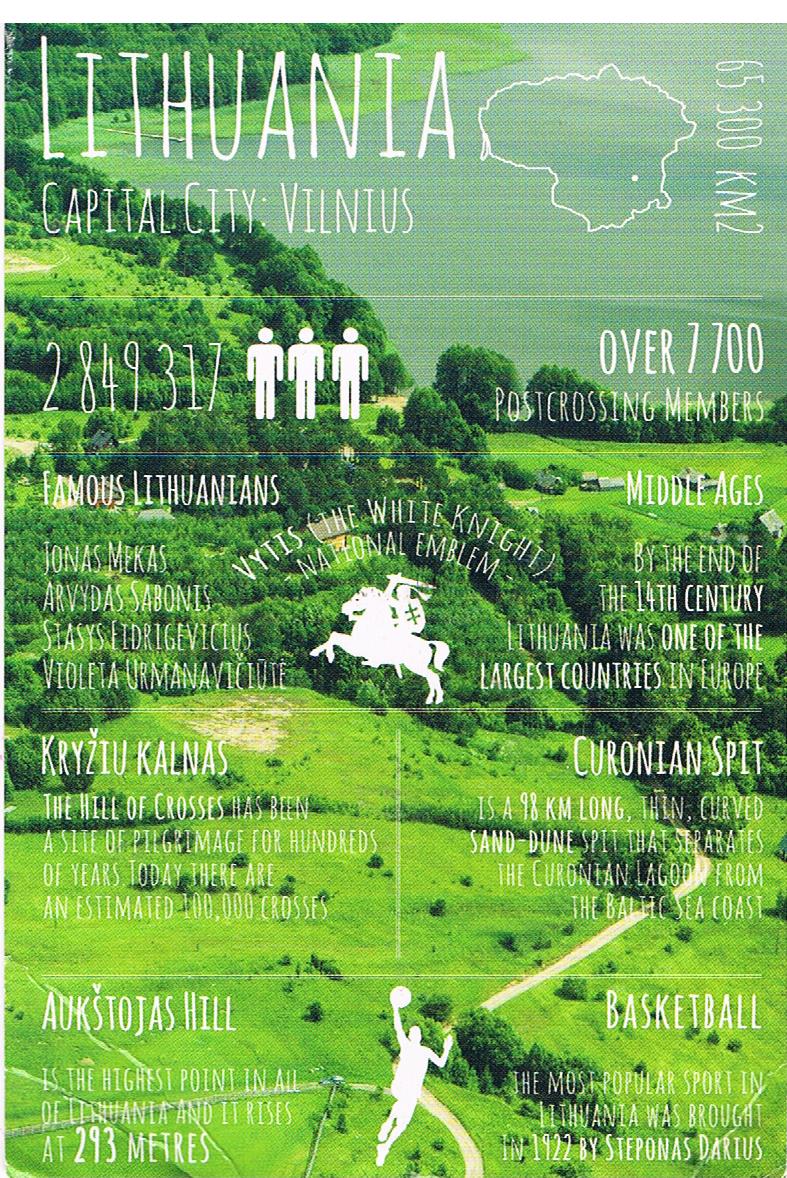The image is an advertisement for the country Lithuania, showcasing its unique attributes and historical facts against a picturesque backdrop. The background features an aerial view of a verdant landscape with rolling hills, lush green fields, and clusters of trees leading to a serene lake. The top third of the image highlights the body of water, while the bottom two-thirds capture the open fields. Superimposed over this natural scenery is white text providing detailed insights into Lithuania.

The text includes the country's name, "Lithuania," and its capital city, "Vilnius." It lists geographic and demographic details such as an area of "65,300 km²" and a population of "2,849,317 people," along with intriguing statistics like "over 7,700 post-crossing members." Historical notes mention that by the end of the 14th century, Lithuania was one of the largest countries in Europe. The image celebrates "famous Lithuanians" including Jonas Mikas, Herbius Sabonis, Satyas Violet, Irman Sivil, and Ivic the White Knight.

Centered on the image are figurines representing people, a horse, and a basketball player, underscoring Lithuania's rich cultural heritage and love for sports. Prominent landmarks such as Križiukalnas, the Kronian Spit, and Aukštosčaš Hill are also mentioned. This advertisement effectively captures the essence of Lithuania, blending its natural beauty with cultural and historical richness.